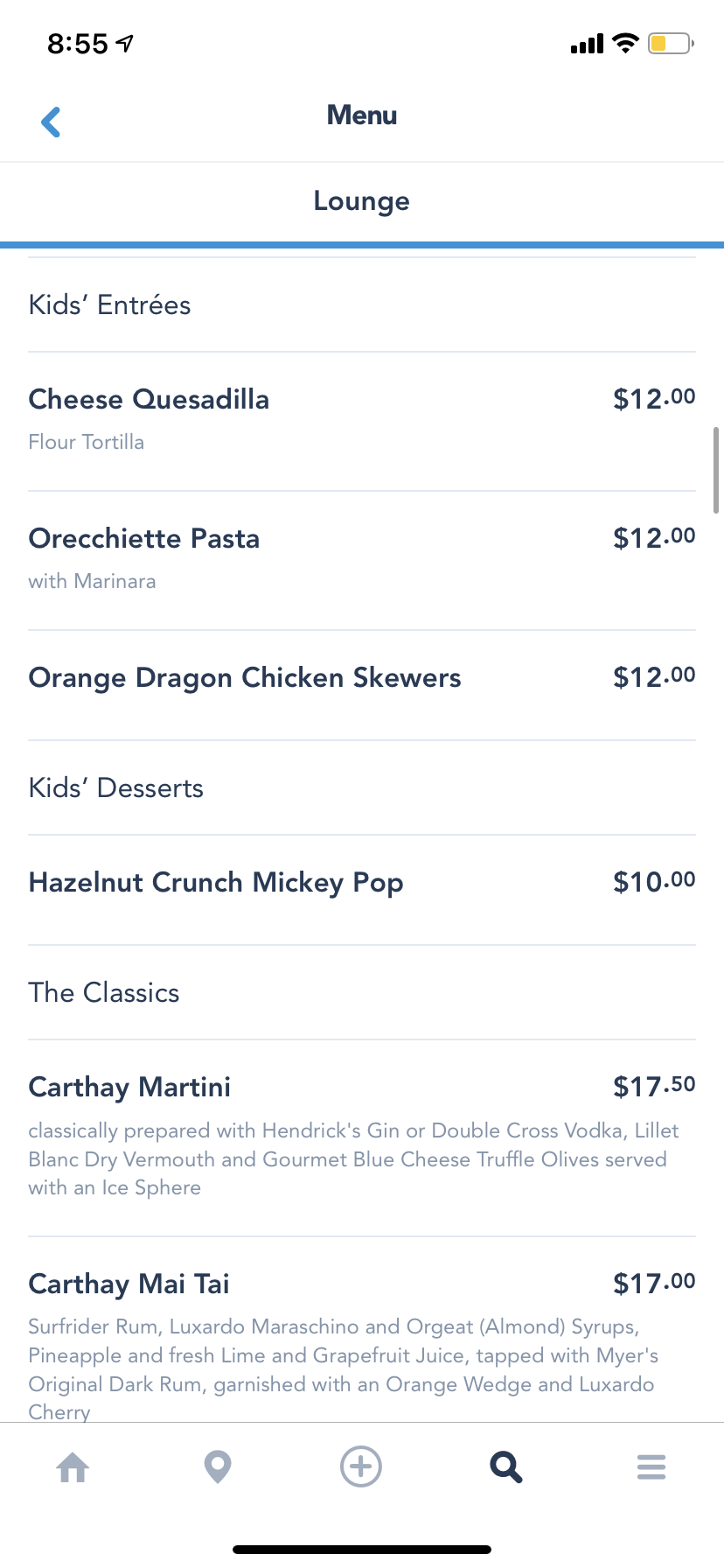The image depicts a minimalistic placeholder graphic set against a pristine white background. At the center of this vast expanse of white space, a minuscule thumbnail icon resides, barely larger than a speck. This tiny marker serves as an indication that an image is intended to be displayed in this location. The stark simplicity and ample negative space emphasize the placeholder's understated presence on the page.